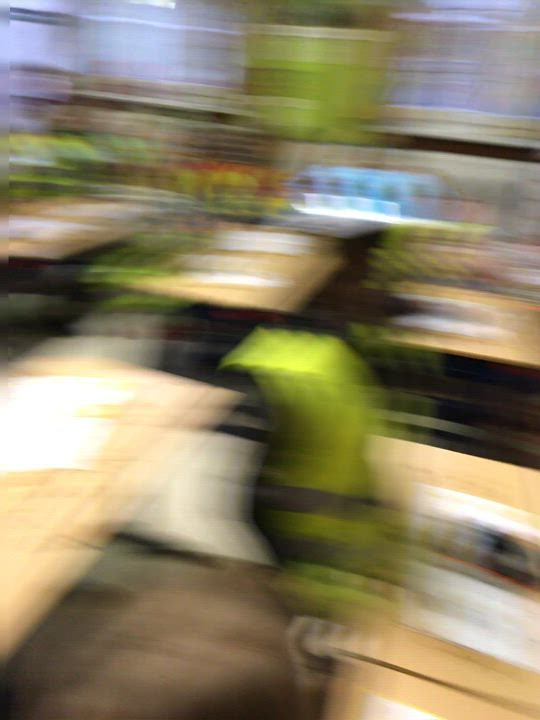In this blurred image, rows of closely arranged desks or countertops stretch into the distance, creating an indistinct yet organized setting. Prominently in the foreground, a vivid acid green-yellow object sits on one of these surfaces, surrounded by white pieces of paper, adding a hint of activity despite the motion blur that suggests either the camera or the objects themselves are in motion. A large, green pillar stands tall in the background, and streaks of white, possibly from rapid movement, add to the chaotic feel of the scene. Additionally, a blue object can be spotted further back, contributing to the array of colors and forms that populate this dynamic, albeit blurry, environment.